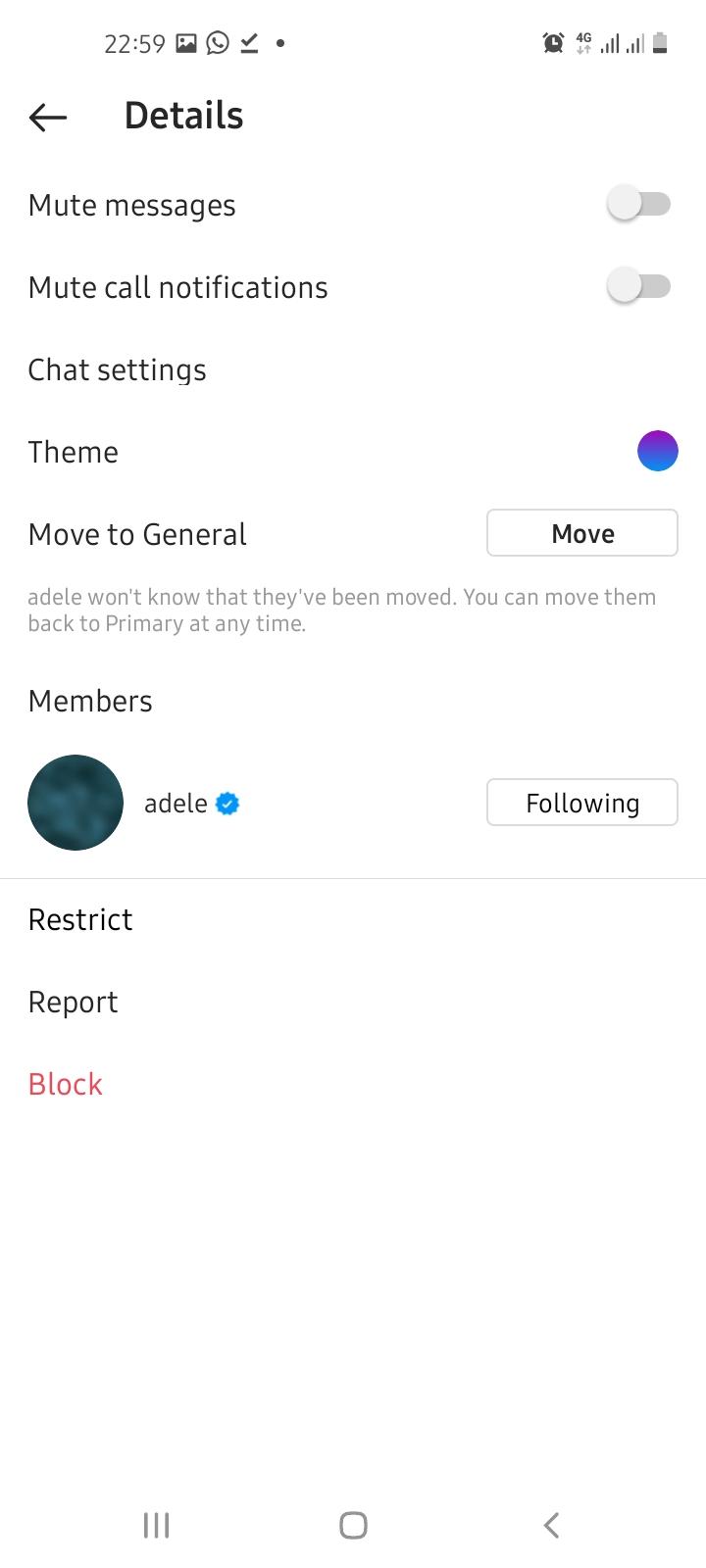**Detailed Caption:**

A detailed screenshot of a control panel on a smartphone, likely from a social media app. The top of the screen displays the current time as 22:59, alongside several icons: an image icon, a WhatsApp icon, a checkmark, an alarm clock, a 4G network indicator, and signal strength bars showing four bars for one signal and three bars for another. The battery icon indicates approximately 20% remaining. To the left, there is a back arrow, and the title "Details" is shown prominently at the top.

Below, the interface includes several toggles and settings. "Mute messages" and "Mute call notifications," both disrupted by 'Off' sliders, are clearly visible. Paying attention to the "Chat settings," an option for "Theme" reveals a bluish-purple selection.

Next to "General," is a move button. An explanatory note below suggests, "Adele won't know they've moved. You can move them back to primary at any time." The "Members" section lists a name, Adele, with a verified blue checkmark and a slightly blurred profile picture. Corresponding buttons include "Following," a grayed-out text "Restrict," "Report," and a red "Block" button.

The screen ends with some white space and the simple navigation menu at the bottom, marked by three distinct buttons. The overall impression suggests this screen pertains to managing a user's contact or interaction settings, possibly on a platform like Twitter.